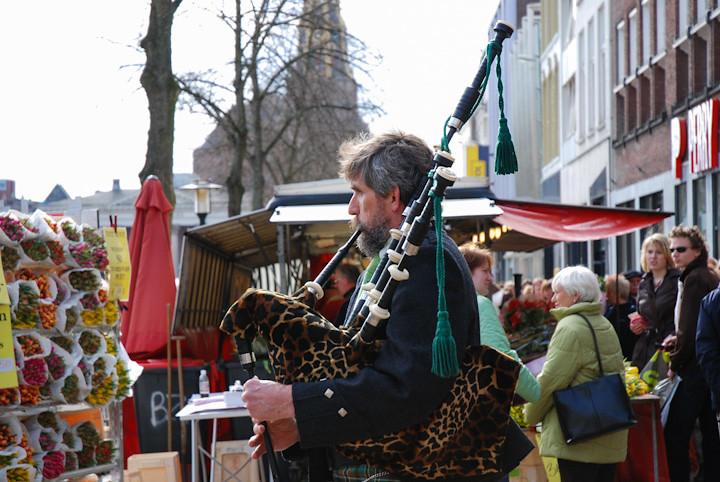In this vibrant daytime photo of an outdoor farmer's market, the central figure is an older gentleman with gray hair and a beard, dressed in a wool navy jacket adorned with buttons on the sleeves. He is playing a bagpipe that features a distinctive leopard print bag with green tassels and black pipes. Surrounding him is a lively scene: in front of him stands a rack overflowing with a variety of colorful flower bouquets, including hues of yellow, orange, rose, and red. Behind him, a flower stand and a food stall are busy with people, many of whom are wearing coats. The background reveals a row of buildings and, towards the upper right, the blurred silhouette of a brick church against a white sky. Amidst the scene, a closed red umbrella and an open red umbrella dot the sidewalk, with tree branches peeking from behind the stalls, adding a touch of greenery to the bustling market environment.